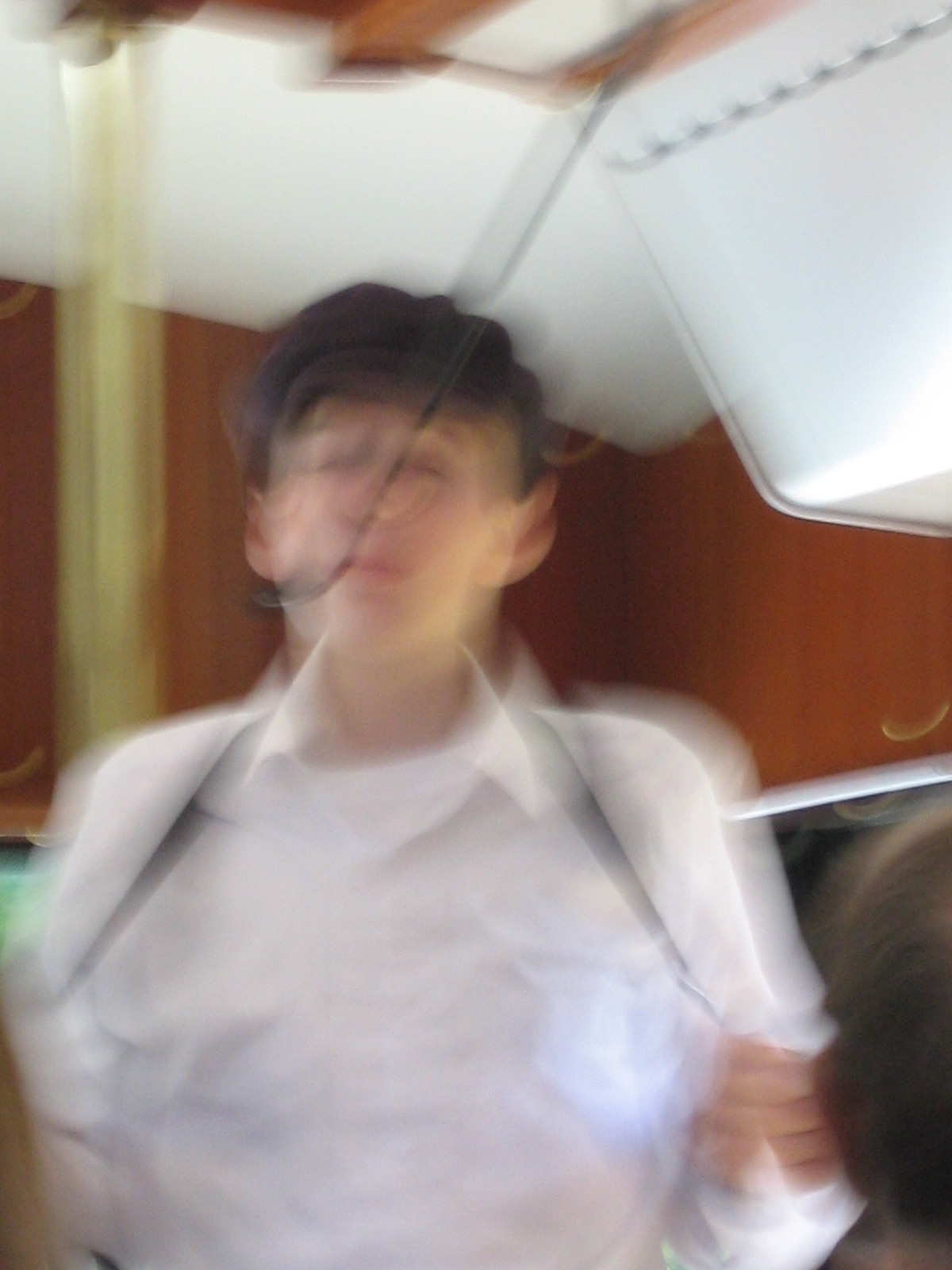In this blurred photograph, a man with dark hair stands toward the left side of the frame, facing the camera head-on. He is dressed in a white button-down shirt with a white t-shirt underneath. A black strap, likely a bag or camera strap, hangs around his neck, with his left hand raised to hold it while his right hand is not visible. On the left side of the image, a light pea green pole descends vertically from the top of the frame. In the top right corner, a white box is suspended in the air, connected to a white pipe that extends horizontally from the left-hand corner into the box.